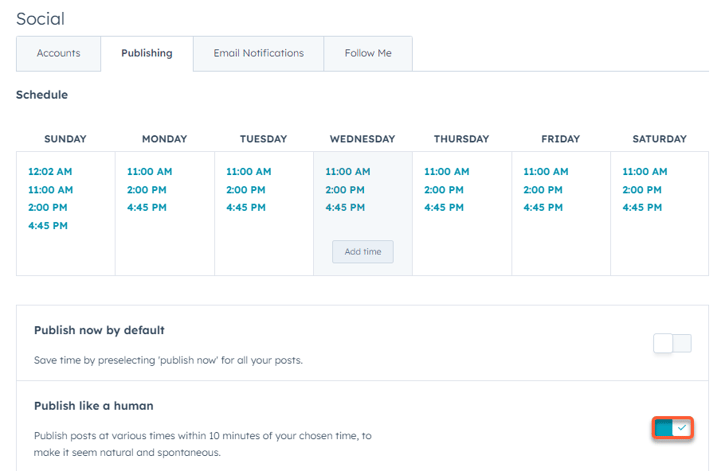The image depicts a social media management interface with a highlighted tab labeled "Publishing." The screen is organized with additional tabs for "Accounts," "Email Notifications," and "Follow Me." The "Publishing" tab reveals a detailed schedule for posting content throughout the week, listing specific posting times: Sunday at 12:02 AM, 11:00 AM, 2:00 PM, and 4:45 PM; Monday through Saturday, the times are consistently 11:00 AM, 2:00 PM, and 4:45 PM, except for Saturday, which includes a 4:45 AM posting as well.

For Wednesday, there's an additional option to add a new posting time. Below the schedule, there are options for "Publish Now" and "Publish Like a Human." The "Publish Now" option is not selected by default. The "Publish Like a Human" feature is enabled, marked by a checked box within a red square. This feature ensures that posts are published at slightly varied times—within a 10-minute window of the scheduled time—emulating a more natural and spontaneous posting behavior.